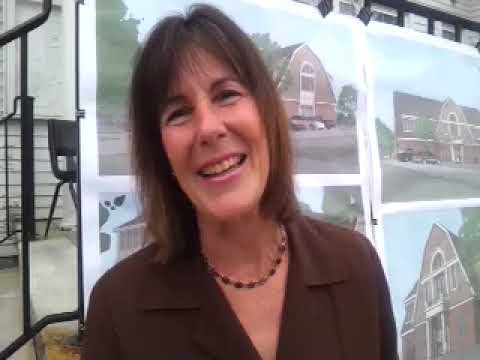A photograph captures a woman of likely Caucasian descent with short, straight, shoulder-length brown hair, accented by darker bangs framing her face. She is dressed in a collared, short-sleeved brown blouse and a simple necklace. The woman's expression suggests she is engaging in conversation; her eyes are partly closed, forming narrow slits, and her mouth is slightly open in a circular shape, possibly indicating she’s mid-sentence.

She stands prominently at the center of the image, with her surroundings providing context. Behind her is a white house with black cast iron railings and a gray staircase. Adjacent to her and slightly to the left is another house in a brown hue, set against a backdrop of blue sky and green grass. A banner featuring various schematic images of houses or perhaps a barn drapes over the railing, suggesting she might be presenting them, possibly in the context of real estate. There is also a single black chair with two openings, positioned near what appears to be a door. The scene appears to be outdoors, possibly during an interview or an informal presentation.